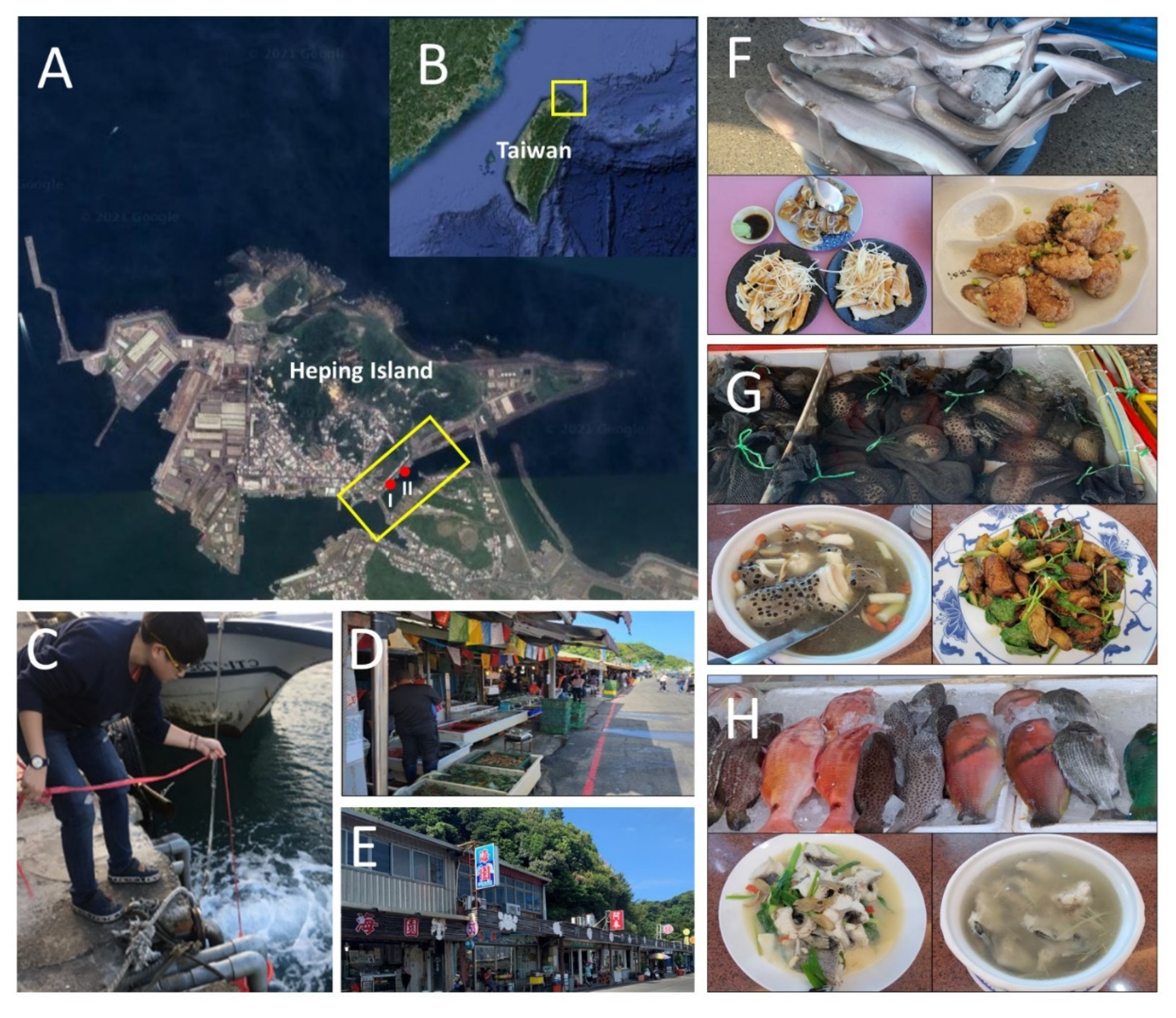This image is a detailed montage of various photographs, primarily focusing on an island and its regional seafood culture. The largest photograph, labeled A, is positioned at the top left corner and features an aerial view of Hepping Island, identified by its text label. Adjacent to it is photo B, in the top right corner, showing an overhead shot of Taiwan with a particular area highlighted in yellow to indicate the location of Hepping Island. Both A and B emphasize the geographic connection between Hepping Island and the highlighted northern region of Taiwan.

Below these, photo C captures a fisherman in the act of pulling a catch from the shore, hinting at the island's fishing activity. To the right of this, photo D depicts a bustling seafood market, rich with fresh catches. Adjacent to D, photo E shows a line of buildings, likely part of the marketplace or surrounding area. Continuing to the right, photo F illustrates a collection of various fish displayed on ice, with accompanying photos of dishes made from these fish, showcasing traditional seafood preparations. Below this, G features images of squids and then transitions into dishes prepared from squid, further highlighting the region's culinary diversity. Finally, photo H at the bottom focuses on what appears to be halibut, along with various cooked dishes made from this particular fish, emphasizing the extensive use of local marine resources in the island's cuisine.